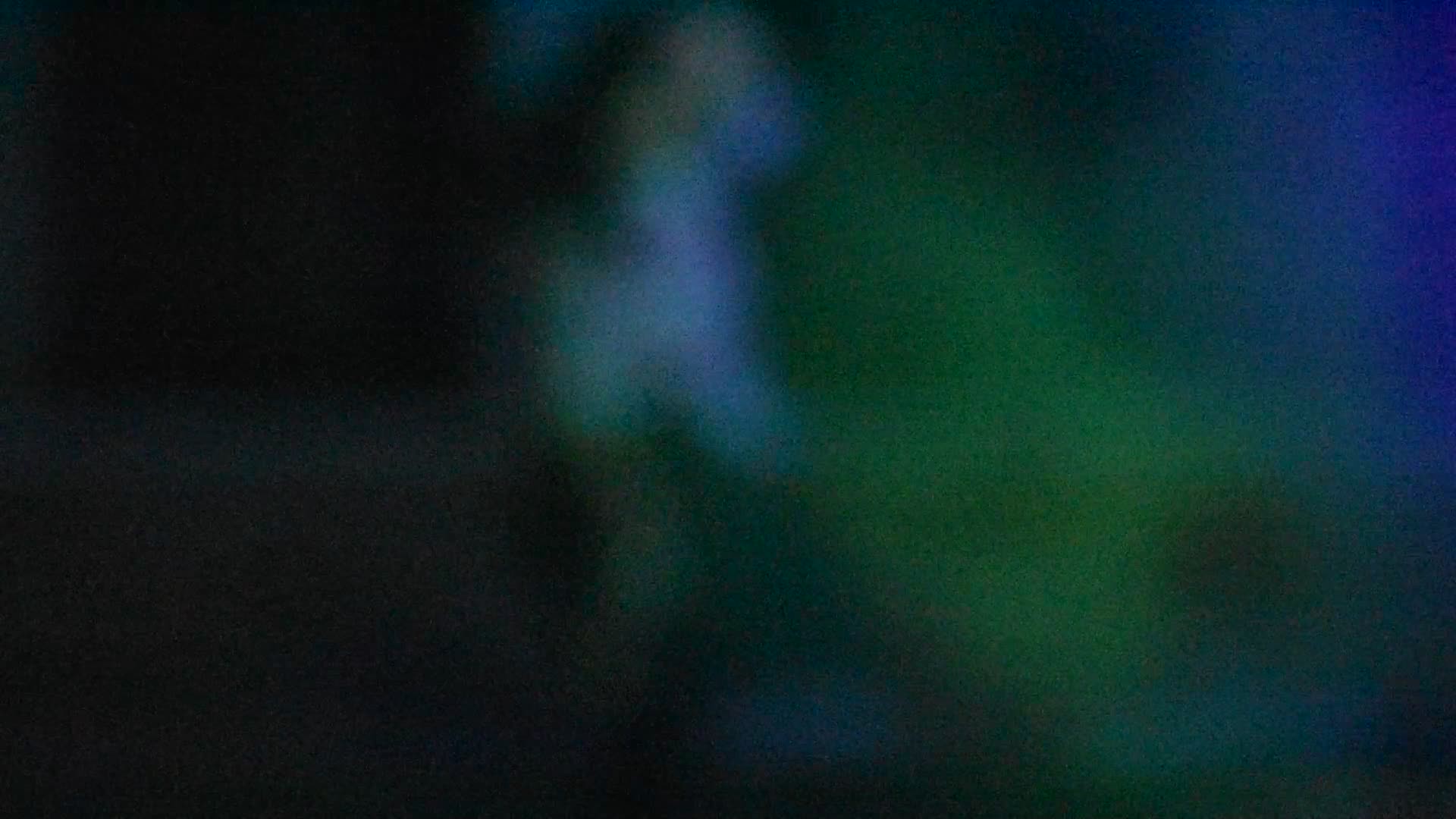This is a very blurry photograph in landscape mode, lacking any discernible shapes due to significant blur and fuzziness. The image predominantly consists of a range of colors: dark black on the upper left corner fading into dark gray towards the bottom right, with a more noticeable blotch of white splotch in the center. To the right of the central white splotch, there's an indistinct green blur that transitions into varying shades of blue moving towards the top right corner. The photograph appears to be taken in a dark environment, perhaps at night or in a dimly lit room, characterized by the prevalence of dark blues and blacks, accompanied by greens and whites. Some interpretations suggest the possibility of a figure or object in the middle area, with mentions of familiar shapes like a My Little Pony or a person in a white coat with light blonde hair. However, these interpretations remain speculative due to the image's extreme blurriness, presenting an ambiguous scene that could be anything from a dark kid's room to an outdoor setting.